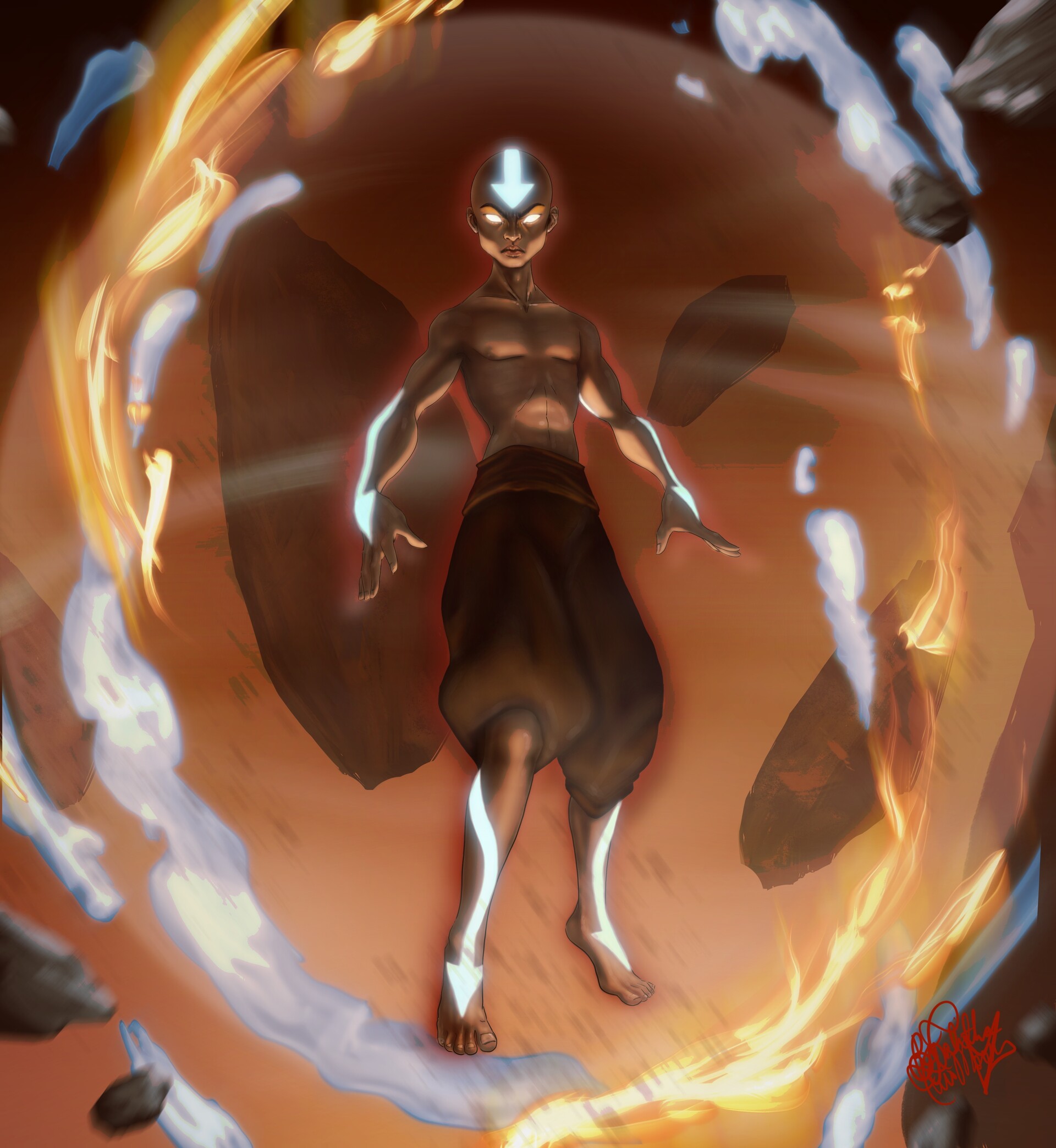The image depicts a highly detailed and dynamic fan artwork of Avatar Aang from the series "Avatar: The Last Airbender." Aang, shown in the powerful Avatar State, is floating mid-air with his iconic arrow tattoos and eyes glowing brilliantly. He appears shirtless, wearing traditional genie-style gaucho pants that reach his knees. The arrows extend down from his bald head to his eyes, and similarly, from his arms and legs. Aang's expression is one of intense focus and anger as he looks down, channeling immense energy. Swirling around him are glimmers of light, clouds, and the four elemental forces: air, fire, water, and earth, symbolizing his mastery of all elements. Rocks seem to be forming or floating around him, reinforcing the theme of elemental control. In the bottom right corner, there is an artist's signature, though it is partially illegible. The scene captures a moment of considerable power and poised fury, reverberating with an ethereal and commanding presence.